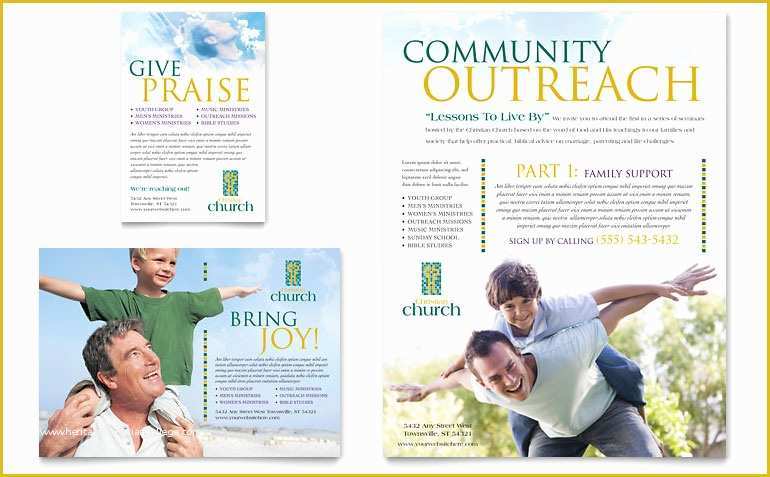The image displays a vibrant collection of three church flyers, each conveying messages of faith and community. In the top left-hand flyer, amidst a sky filled with clouds and a blend of blue hues, a man's face is transparently superimposed, gazing upwards towards the prominent text "give" in green and "praise" in large yellow letters. Below this message is a list of bullet points in dark purple-brown, followed by an illegible paragraph, and finally the word "church" in the bottom right-hand corner. The church’s logo, a yellow-outlined cross against a green pattern, is also present. 

The bottom left-hand flyer captures a heartwarming scene of a Caucasian man with dark hair, wearing a white shirt, carrying a joyful young blonde boy with a green shirt on his shoulders. The text "bring joy" in green and yellow enhances this uplifting image, which features a blue sky background and the church logo in the top right corner. The accompanying text is too small to read clearly.

The right-hand flyer is significantly larger, spanning from the top to the bottom of the image, with the words "community" in green and "outreach" in yellow at the top. This flyer includes a paragraph titled "part one" in yellow and "family support" in purple. It features a man wearing a white shirt and gray pants, bent over with his arms outstretched, carrying a child with dark brown hair in a light blue shirt on his back, both mimicking a playful airplane pose. The backdrop shows lush green trees, and the church logo is positioned near the boy's head on the left. The entire composition is bordered in gold, giving it a cohesive and polished presence.